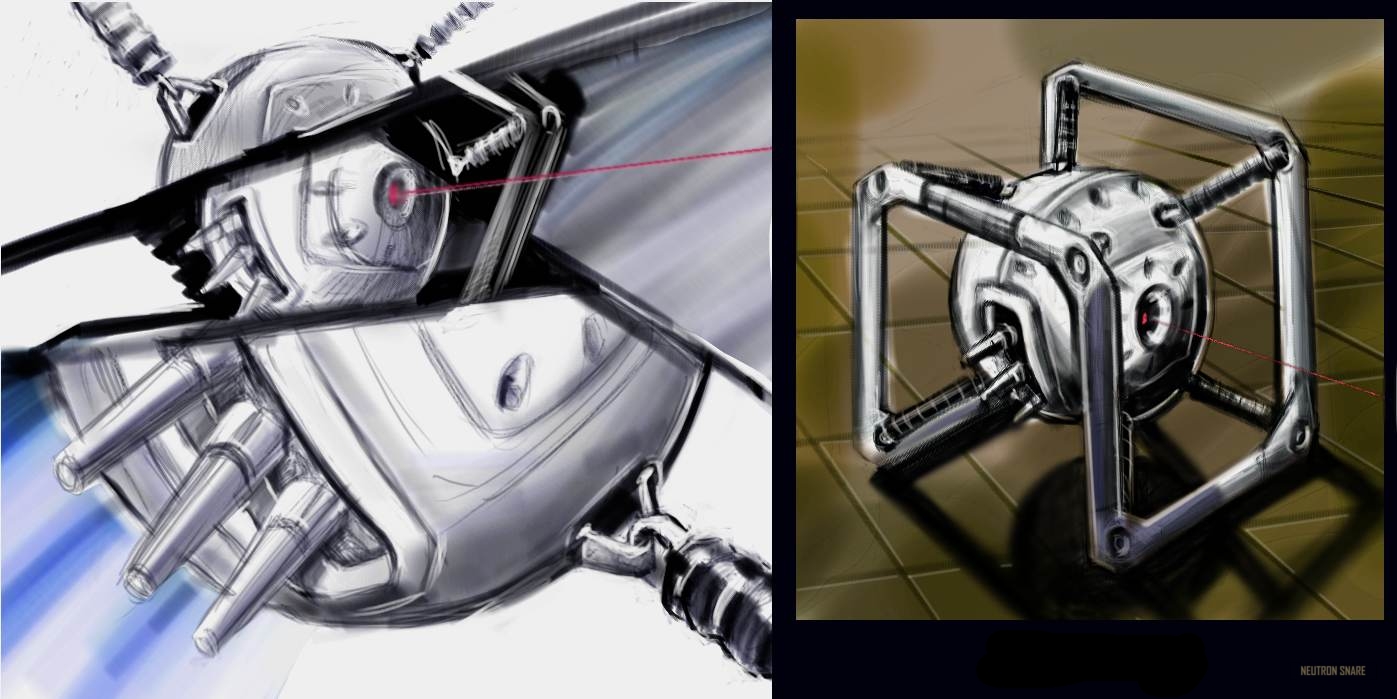In this detailed illustration, two side-by-side cartoon drawings depict a futuristic robot with advanced technology. The robot is a square-shaped contraption featuring a spherical component attached to its cube-like body. In the image on the left, a vivid red laser beam is shown projecting from the robot's eye-like feature, demonstrating its capability to emit powerful laser beams. This technological marvel appears to be both sophisticated and somewhat ambiguous, with lights and beams shining out, enhancing its advanced appearance. Despite the overall clarity of the robot's function, the context or the specific cartoon series to which it belongs remains unknown. The right-side image also illustrates the robot shooting a laser beam, though it appears from a more distant perspective, providing less detail. This highly intricate artwork showcases the robot's striking technological design and its laser-emitting capabilities.